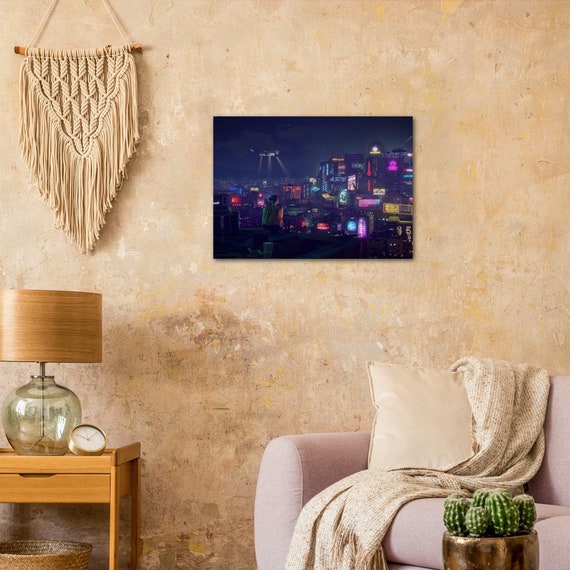The photograph depicts a cozy living room with muted and earthy tones, featuring a wall with a patchwork of colors including tan, yellow, white, and light brown. Dominating the bottom right corner is a very light tan-colored couch adorned with a white pillow and a light brown blanket. In front of the couch sits a planter with various green cacti, housed in a dark golden bowl. The bottom left corner showcases a light brown table with a matching lamp and a small golden clock with a white face beside it. Hanging on the top left section of the wall is a beige macrame tasseled artwork. The centerpiece, however, is an unframed nightscape painting in the middle of the wall depicting a city skyline with vibrant hues of blue, pink, and purple, featuring a floating object illuminated by beams of light from below.